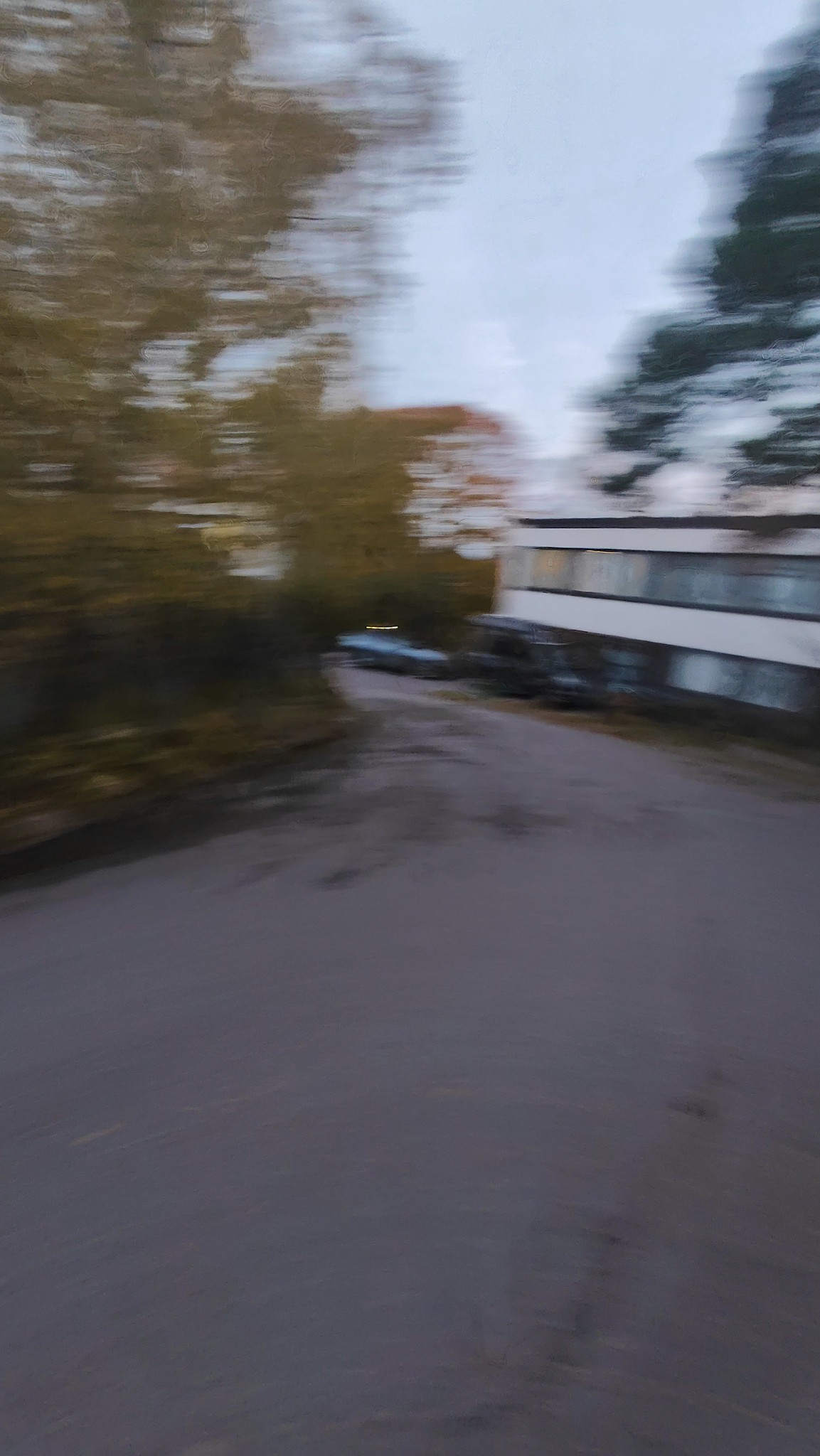This photograph depicts a blurry, motion-blurred image of a blacktop neighborhood street that curves left in the distance. On the right side of the street stands a modern white house with a black trim. The house features a row of glass windows at the top and two large windows at the bottom. In front of this house, there are two parked vehicles: a large black van and a smaller blue car. Surrounding this area, tall, deep green trees extend over the rooftops. On the left side of the image, partially obscured by trees and motion blur, there appears to be another house or structure, potentially yellow in color. The left side foreground includes bushes and a group of trees with yellowish-green foliage. The street itself shows some dark patches, which could indicate potholes developing.